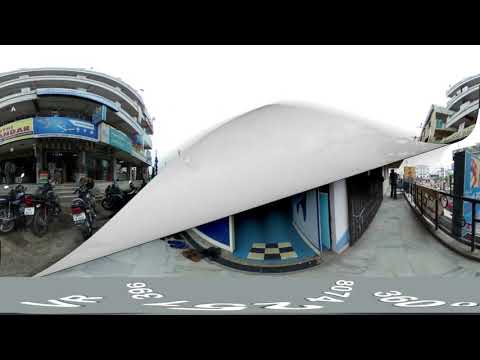This digitally-created photo, possibly extracted from a video flipping through images, captures a curved four-story building on the left, adorned with colorful signs in yellow, blue, and green. Several black motorcycles are parked at its gray front steps, facing the entrance. The image features a 360-degree view framed by horizontal black bars at the top and bottom. A notable element is the effect of a white page corner being flipped upward, revealing a new scene underneath. This revealed section presents another curved building with a bright blue interior, a black-and-white checkered square in front, and a gray paved walkway with black rails. A person stands in the far distance of this surreal, day-lit scene. The text "VR257" is visible at the bottom of the screen, further suggesting a digitally altered or virtual reality composition.